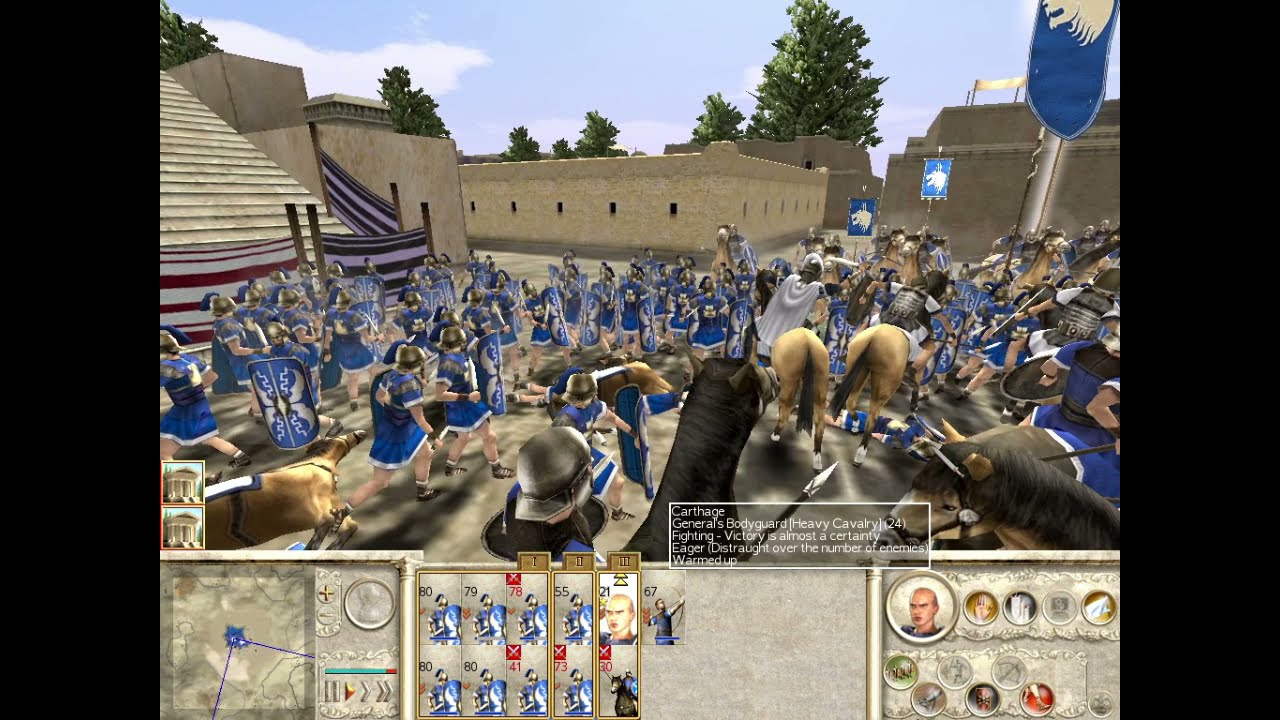The image is a screenshot from a video game depicting a medieval battle scene within a castle setting. It features a large group of soldiers, some on horseback and others on foot, all clad in blue uniforms with metal helmets and silver-blue shields. They are lined up and appear to be preparing for battle. Blue banners, partly obscured but seemingly adorned with a white lion or wolf, are visible among the troops. The backdrop includes grayish light brown buildings, a stairway to the left, and a clear blue sky with scattered clouds. Trees dot the distant background, adding to the scene's depth. Numerous horses, some seemingly fallen, are scattered throughout the melee. At the bottom of the screen, video game controls and icons for troop selection, the general, and the map interface are displayed.